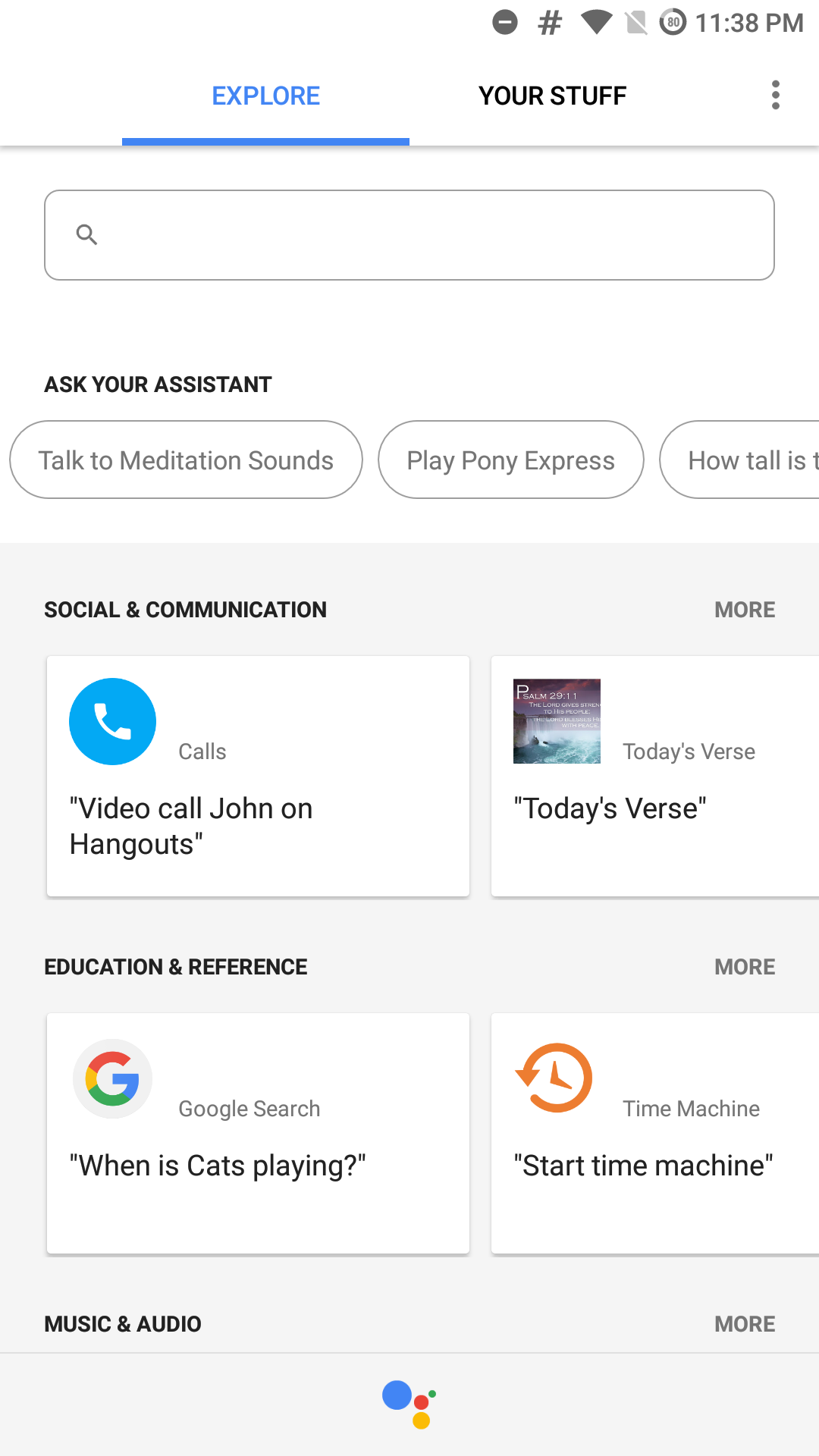A screenshot of a modern smartphone display is shown. At the very top, a few status icons are visible, indicating that the Do Not Disturb mode is enabled. Following that, there is a hashtag symbol whose specific purpose is unclear but might be related to social media applications such as Twitter or X. The Wi-Fi symbol follows, showing an active connection, while an icon suggests that there's no SD card inserted. The current time "11:38 PM" is displayed prominently.

Below these status icons, the screen displays what seems to be an open Google Assistant interface, specifically in the "Explore" tab. To the right of the "Explore" tab is another tab labeled "Your Stuff," which can be selected. There are three vertically aligned dots next to these tabs, likely indicating additional options or settings.

Beneath the tabs, a search bar is labeled with the prompt "Ask your assistant," followed by several suggestions including "Talk to meditation sounds," "Play Pony Express," "How tall is..." with the remainder of the suggestion cut off. Below these suggestions are categories such as Social, Communication, Recommendations, Education, and Reference, offering various ways the user might utilize the Google Assistant. Overall, the screenshot captures a comprehensive look at the Google Assistant homepage, showcasing suggested uses and categories for user interaction.